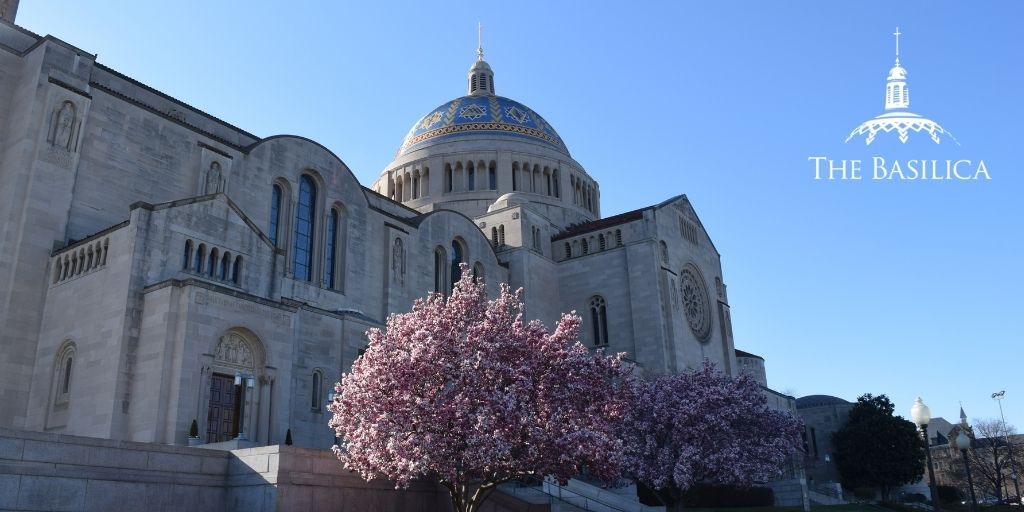This is a detailed daytime photograph of the Basilica, captured from ground level looking upward, with a clear blue sky providing a vibrant backdrop. The building is a grand, light gray stone structure, reminiscent of an old cathedral, featuring multiple tall, narrow, arched windows and inlays of statues in the exterior walls. The Basilica's facade includes massive wooden doors situated on the left side, partially obscured by two lush cherry blossom trees in full pink bloom, and flanked by at least two street lamps with white covers.

The most striking feature of the Basilica is its large central dome, which is ornately decorated in blue with gold, red, and yellow detailing. Surrounding the base of the dome are small windows, and rising from its top is an elegant cupola and a spire, crowned by a cross. Additionally, there is a circular window and columns that add to the building’s intricate design.

In the upper right corner of the photograph, the word "Basilica" is written in thin white text alongside an emblem depicting the dome and cross, enhancing the formal identification of this impressive structure.